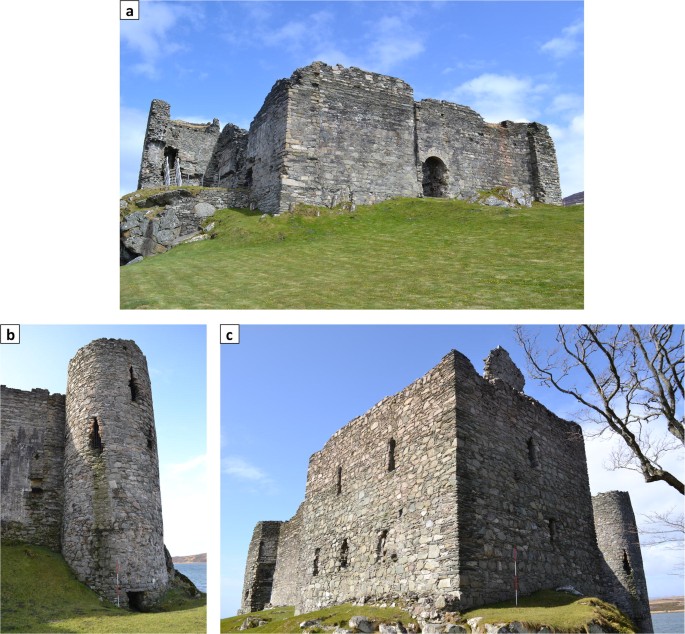The three images depict different angles of Castle Sweene located in Scotland, showcasing its ancient, grey stone architecture against a backdrop of blue skies, white clouds, and lush green grass. Image A at the top captures a frontal or rear view of the castle featuring a large, decrepit arched doorway at its center, with an extension that seems to house a chimney and a ladder. Image B, positioned at the bottom left, highlights the castle's round turret with three window openings—two at the top and one at the bottom—stood next to the water, possibly a lake. Image C on the bottom right displays a broader view, revealing the corner of the castle. It features a sharp angle with multiple window openings; the left side has two windows on top and three on the bottom, merging into the rounded turret seen in Image B. The castle, thought to be centuries old, appears fragmented and weathered, with its differing shades of grey stone and missing roof, conveying a sense of historical grandeur.